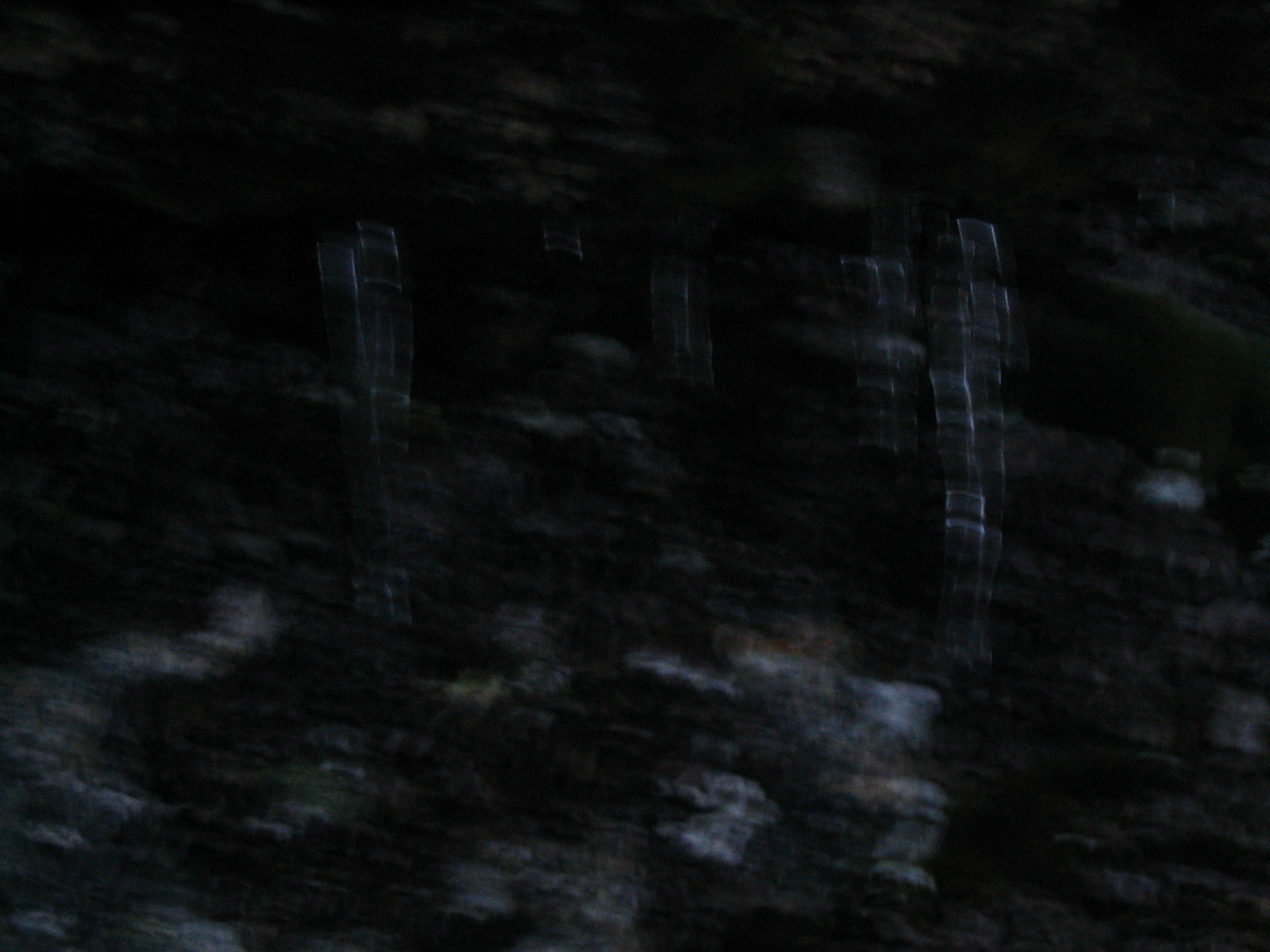This extremely blurry and dark photograph, rectangular in shape, depicts an indistinct outdoor scene taken at night, possibly from a moving vehicle. The image is dominated by black and gray hues with sporadic patches of white and light gray. The background features long, vertically oriented shapes that could be the silhouettes of trees or posts anchored into the ground. In the lower left corner, the tiny white patches seem almost cloud-like, emerging from the darkness. Midway through the image, there are white blotches that resemble abstract, ghost-like forms with wavy arms, adding an eerie, ominous feel to the photograph. In the upper right, a vertical trail of light hints at a waterfall cascading over what could be rocks. The photograph's abstract nature makes it difficult to discern details, but elements of rock colors, such as dark brown and light gray, contribute to the overall mysterious and surreal atmosphere.